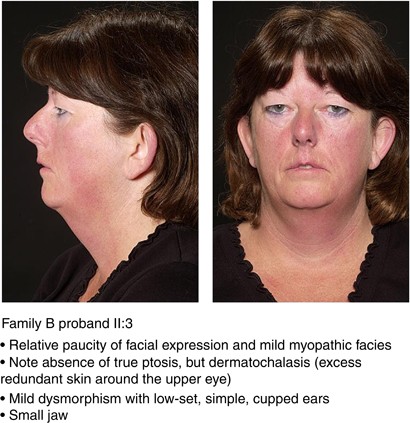The image consists of two side-by-side medical photographs of a middle-aged Caucasian woman with dark brown shoulder-length hair. The left photograph shows her in profile facing the left side, while the right photograph captures her head-on, looking directly at the camera. She is wearing a black V-neck top in both images. The text description underneath identifies the subject as "Family B Proband, 2 to 3," and highlights various medical observations. These include a relative paucity of facial expression, mild myopathic facies, dermatocolisis—characterized by excess redundant skin around the upper eyes—heavily lidded eyes, low-set, simple cupped ears, and a small jaw. These features suggest mild facial dysmorphism, potentially indicative of an underlying syndrome.